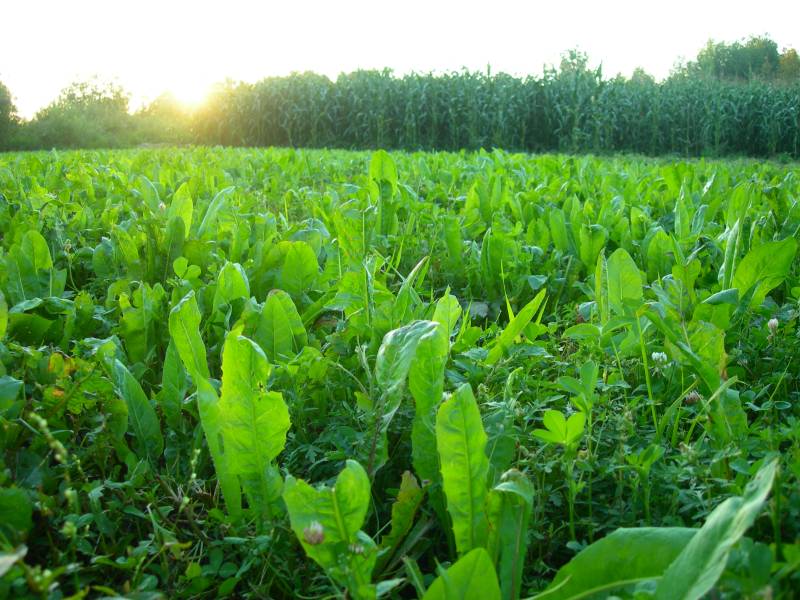The photograph captures an expansive field dominated by various shades of green. In the foreground, a dense mix of weeds and grasses, possibly including dandelions and clovers, proliferates. These plants, featuring leaves approximately 10 inches tall, create a tapestry of light and dark green hues. Interspersed among the vegetation are small white weeds, adding a speckled texture to the ground cover. Midway through the photo, the same types of plants—grasses and weeds—continue to spread across the field. In the distance, a distinct shift occurs as rows of tall corn stalks, characterized by their straight, thin stems and sprouting leaves, stretch towards the sky. The background reveals a row of trees and a partially cloudy sky. The sun, positioned low in the horizon, suggests either a sunrise or sunset, casting a golden glow through the corn and illuminating the scene with a soft light. The entire landscape, from foreground to background, displays a vibrant and varied greenness, anchored by the contrasting textures of the weeds and the structured rows of corn.